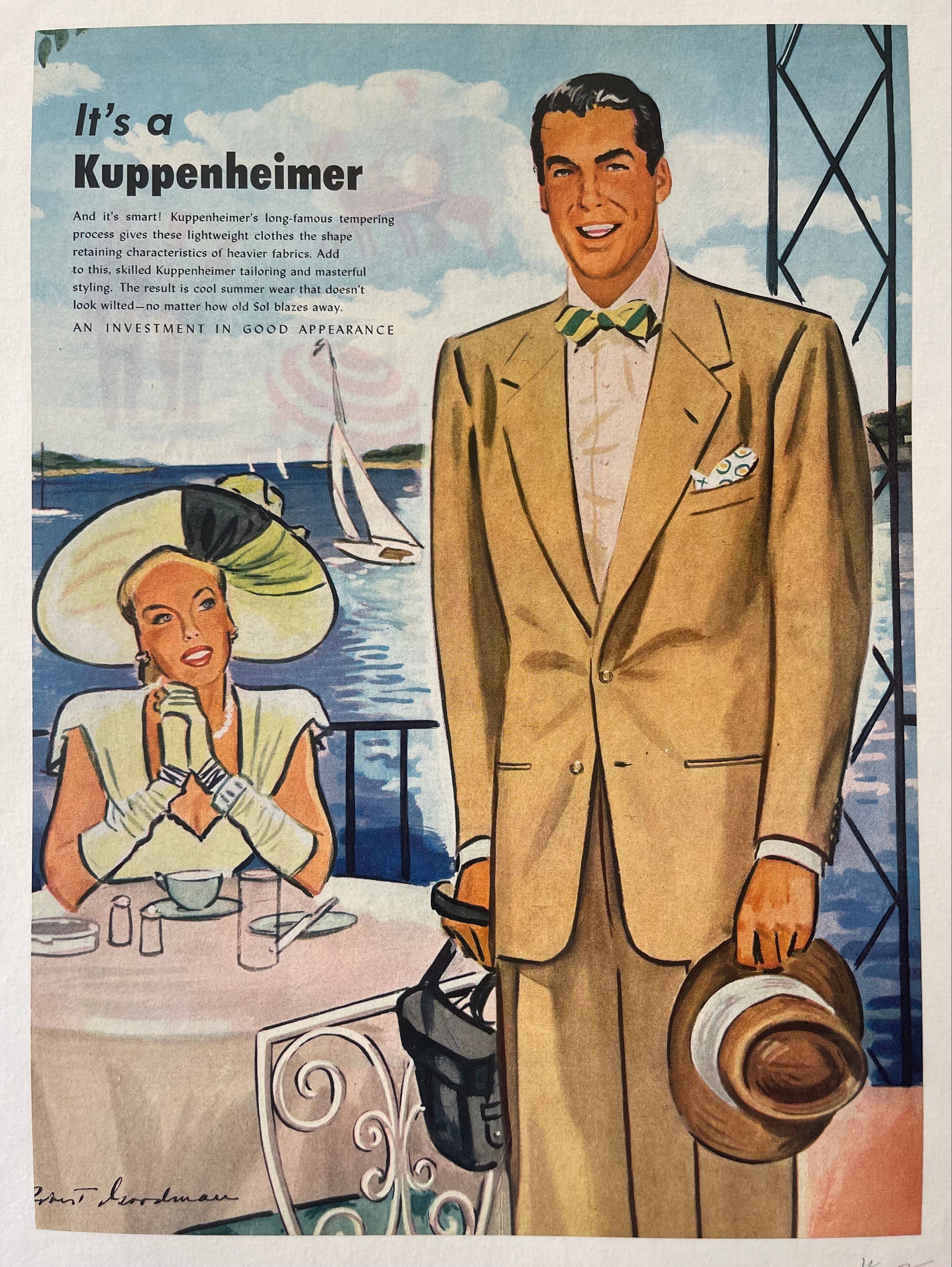The image is a vintage-style advertisement illustration, likely from the 1940s or 1950s, showcasing the sophisticated fashion of the era. At the forefront stands a man in a tan suit holding a white hat with a ribbon in one hand and what appears to be a camera bag in the other. He is adorned with a yellow and green bow tie. Behind him, a woman sits gracefully at a table set with a coffee cup, a teacup, salt and pepper shakers, and a plate. She wears long gloves that reach her elbows and a wide-brimmed white hat with green accents, gazing at the man with admiration. In the background, there is a picturesque view of water with a sailboat, under a blue sky dotted with white clouds. The top of the image prominently features the brand name "Kuppenheimer" with the tagline “It's smart,” followed by a detailed description of their lightweight, shape-retaining summer wear. The ad emphasizes the investment in good appearance, proclaiming that Kuppenheimer’s tempering process and masterful tailoring result in stylish attire that remains crisp even in the blazing sun. The bottom left corner bears the signature of artist Robert Goodman.